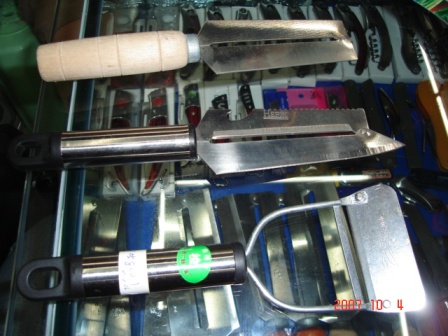The image features three metal tools with plastic and metal handles, resting on a glass-topped display case. The display case contains various packages of different products such as knives and scrapers. Each tool is photographed from the side view. 

The topmost tool has a tan-colored handle with silver metal sides forming a fork-like shape and a gap in between. The middle tool has a silver metal handle and a similar silver forked design, featuring a sharp or serrated edge. The bottom tool has a black plastic handle with a round end; it extends into a structure with two thin dark silver metal rods attached to a flat base. Just above this tool, there are pieces of white and green tape around the handle, along with two silver hooks forming a U-shape and mounted onto a flat silver piece with a small gap. 

The background of the image shows multiple small boxes, predominantly white and silver in color, situated inside the glass display case. These descriptions suggest that the tools might be kitchen or gardening implements, possibly used for peeling, shredding, or cleaning.